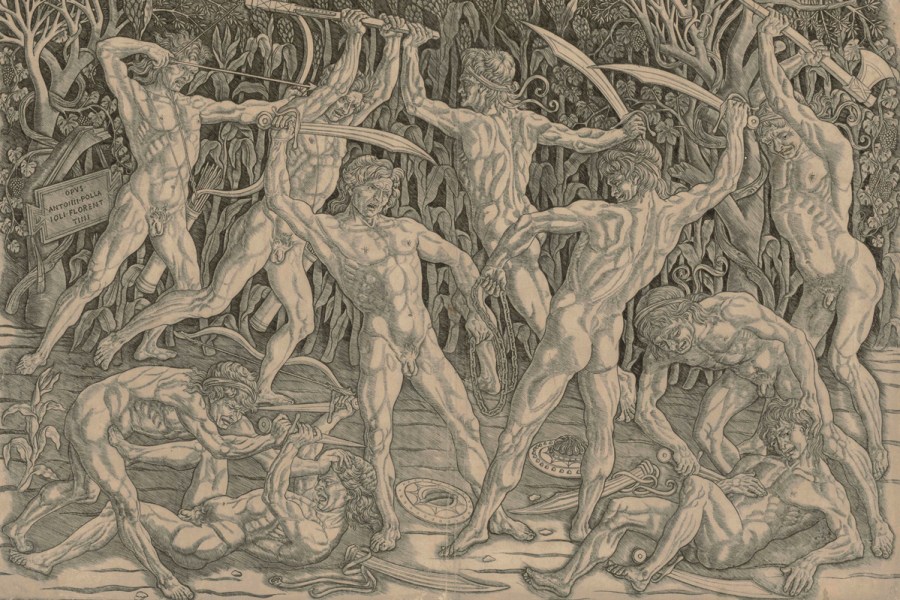This detailed landscape illustration, reminiscent of ancient Greek or Roman style, is rendered in washed-out shades of gray, black, and light brown. It depicts a chaotic battle involving perhaps ten naked men, their muscles meticulously exaggerated through apparent charcoal or pencil shading. The scene exudes intense violence and movement, with men aggressively engaging each other using swords, an axe, a bow and arrow, and daggers. On the ground, several men are involved in close combat; two pairs tussle on either side, while one individual on the right appears to be stabbing another. Fallen weapons and shields scatter the ground. In the background, trees add depth to this highly detailed and dynamic artwork, which notably lacks any text.